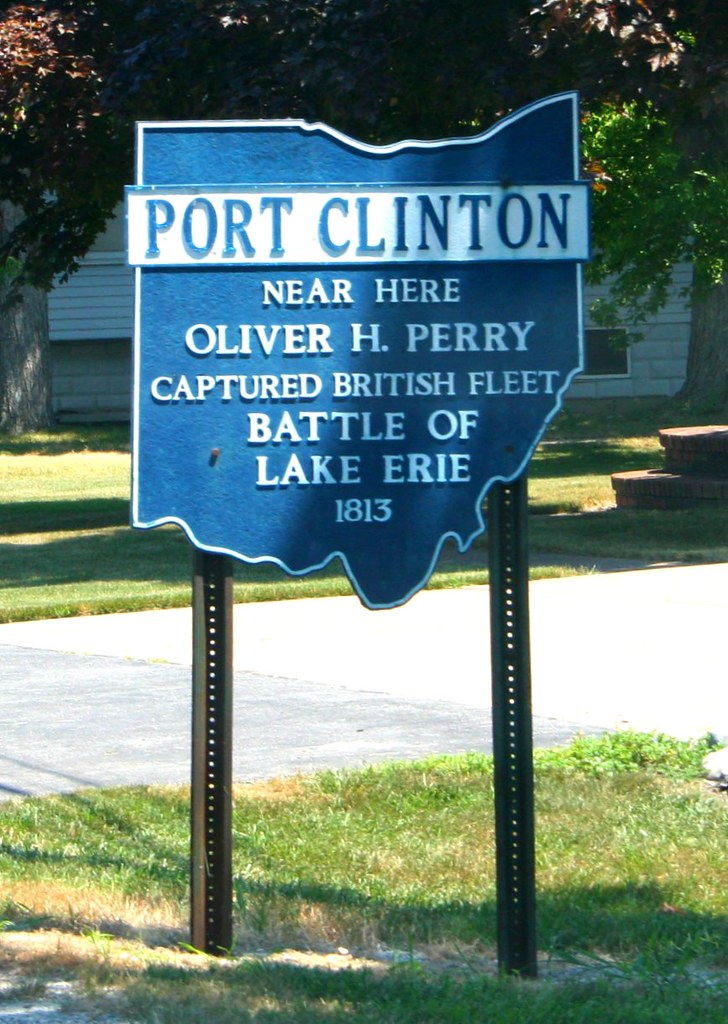In the photograph, there's a blue sign in the shape of the state of Ohio, standing on two metal stilts fixed into the grassy ground. The sign prominently features a white banner at the top with the words "Port Clinton" in blue lettering. Below this banner, the sign reads, "Near here, Oliver H. Perry captured British fleet, Battle of Lake Erie, 1813" in white letters. The setting appears to be a quiet city street, possibly a residential area, with a modest suburban road running through the middle of the grass. A home is visible in the background, partially obscured by trees, and the angle of the shadows on the ground suggests that it is late afternoon. Sunlight is shining directly onto the sign, highlighting the Port Clinton area.